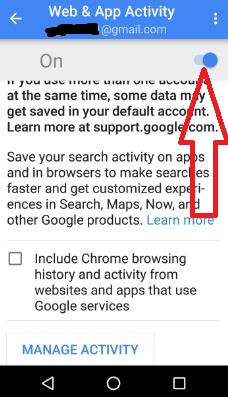The image displays a Google settings interface for web and app activity, associated with a specific Gmail account, though the email is obscured with black. The top section has a blue background with a vertically aligned three-dot options menu in the top right corner and a prominent button on the top left. The content below features a gray background with a highlighted blue toggle switch indicating that the activity tracking is ON. A red arrow points to this toggle switch.

The main body of the text on the white background states, "Save your search activity on apps and in browsers to make searches faster and get customized experiences in search, maps, now, and other Google products." There are links to "Learn more" (in blue text) about data saving and activity settings.

Further down, there is an unchecked checkbox labeled "Include Chrome browsing history and activity from websites and apps that use Google services." Finally, the text at the bottom features another blue link under the gray background, saying "Manage activity," inviting deeper engagement with the settings.